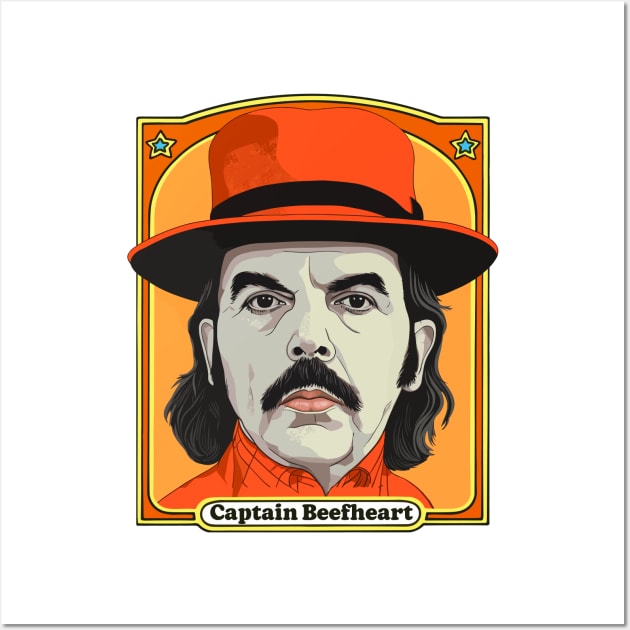The digital drawing features Captain Beefheart at its center, set against a white background framed with an orange border. The border includes two light blue stars, one in each top corner. The focal point is the detailed portrait of a man with bluish-gray skin, pink lips, a large bushy black mustache, and long black hair that reaches his shoulders. He wears an orange collared shirt and a distinctive orange hat with a black underside and a black band around it. At the bottom of the image, a white circle bears the name "Captain Beefheart" in black letters. The man gazes directly forward, creating a sense of direct eye contact with the viewer.